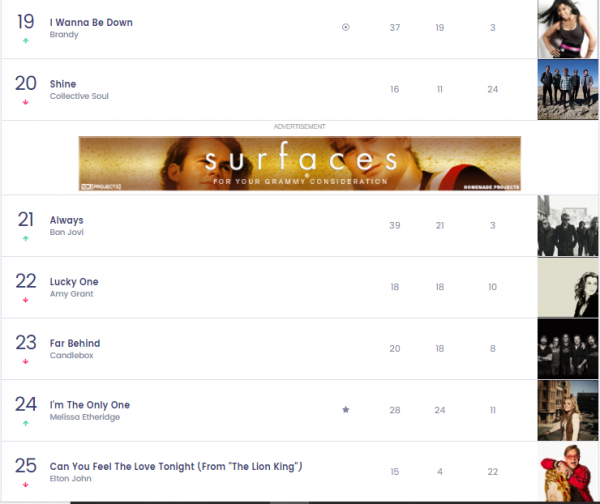The image depicts a table ranking various songs, with entries numbered from 19 to 25. The table has a white background and features text in a gray-blue color. The songs listed appear to be older tracks, though it is unclear if this ranking is official or fan-made.

Here are the details of the songs and their rankings as displayed:

- Rank 19: "I Wanna Be Down" by Brandy.
- Rank 20: "Shine" by Collective Soul.
- Rank 21: "Always" by Bon Jovi.
- Rank 22: "Lucky One" by Amy Grant.
- Rank 23: "Far Behind" by Candlebox.
- Rank 24: "I'm the Only One" by Melissa Etheridge.
- Rank 25: "Can You Feel the Love Tonight?" from *The Lion King* by Elton John.

The table includes various columns with statistical data, although the specific meanings of these numbers are not provided. To the far right, there is a column displaying random photos of the artists rather than their album or single covers. Arrow symbols in green or blue are present beneath the numbers, indicating changes in ranking positions.